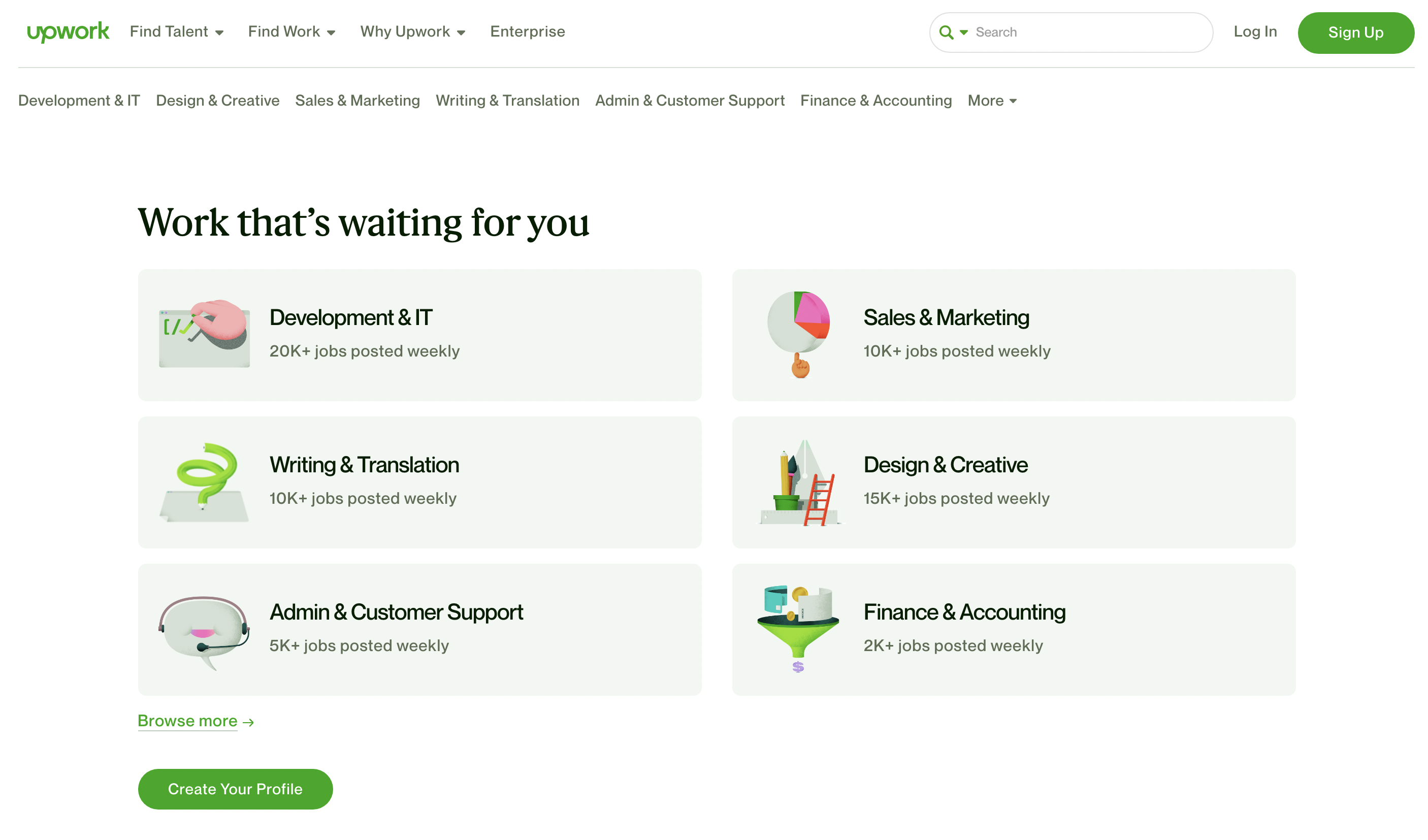The web page depicted features a pristine white background and prominently belongs to the Upwork website, indicated by the Upwork logo in green situated at the top left corner. Adjacent to the logo, there is a primary navigation menu with items displayed in dark blue text. Moving towards the right, the top navigation bar includes a search box, followed by the options to "Log In" and a green oval button with light-colored text that reads "Sign Up."

Below the top navigation bar, another menu is present, leading into the main content area. Dominating this section, in large black letters, is a headline that reads "Work That's Waiting For You." Beneath this message are six distinct light blue rectangles arranged in a grid format—three on the left and three on the right—each featuring a specific category of job listings. 

The top left rectangle is titled "Development and IT" and includes an image of a hand, symbolizing tech-related jobs. Directly below it, the second rectangle is labeled "Writing and Translation," accompanied by a distinctive curly question mark in green. The third rectangle on the left is for "Admin and Customer Support," shown with an icon of a bubble and a headset. Beneath these sections, in green text, is the prompt "Browse More" and a green oval button reading "Create Your Profile."

To the right of these, three more rectangles highlight additional job categories. The top right rectangle reads "Sales and Marketing," followed by "Design and Creative" in the middle, and "Finance and Accounting" at the bottom, completing the grid of job categories presented on the page.